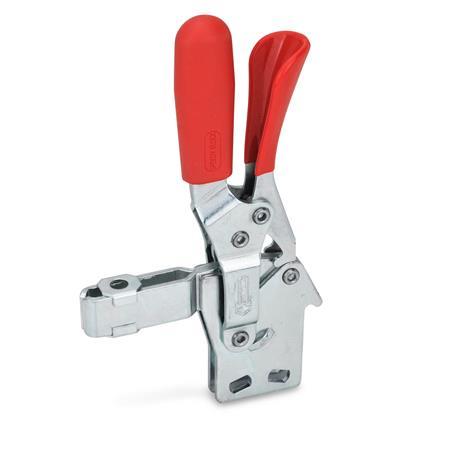This image depicts a fancy can opener-like tool, emphasized by its prominent red silicone handles and high-quality stainless steel construction. The tool, which appears to be upside down and standing on its end against a completely white background, features silver metal components with intricate details. The two bright red handles are designed for squeezing together, with hinges connecting them to a square base. This base includes various mechanisms: on the right side, about halfway up, there is a flared edge intended to hook into cans, and on the left, a small rectangular protrusion with a circular feature on top. Additionally, the bottom of the tool shows two small, dark gray rectangles angled at 45 degrees, possibly for additional functionality. One handle has a visible print label, though it's not legible, adding a touch of branded detail to this sleek, complex contraption that appears fit for online shopping.